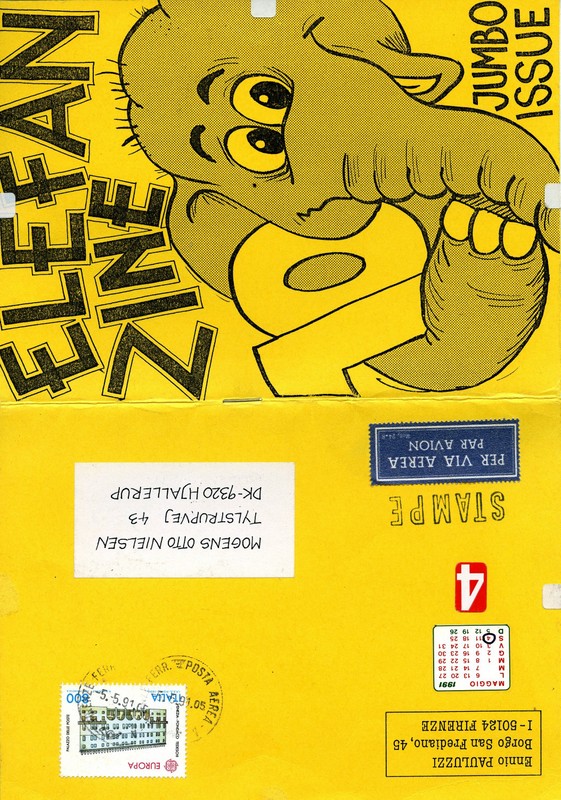The image features a postcard, or possibly a magazine or zine, that's tipped over on its vertical axis, making the bottom part appear horizontal and upside down. The postcard has a yellow background with various postmarks and stamps. The recipient's address, though partly obscured and difficult to read due to its upside-down orientation, includes details like "modus auto Nelson tile Sarupa J 43 DK 9 3 2 0 H Jallerup" and "In Nuri Paul Palazuz Barrago San Ferndino 45 I-5 0 1 2 4 FIRENZE." There's a prominent illustration on the right side of the postcard featuring a gray elephant holding the number 10 with its trunk. Above the elephant image, the text "ELEFAN ZINE" is written, and in the lower right-hand corner, it says "JUMBO ISSUE."